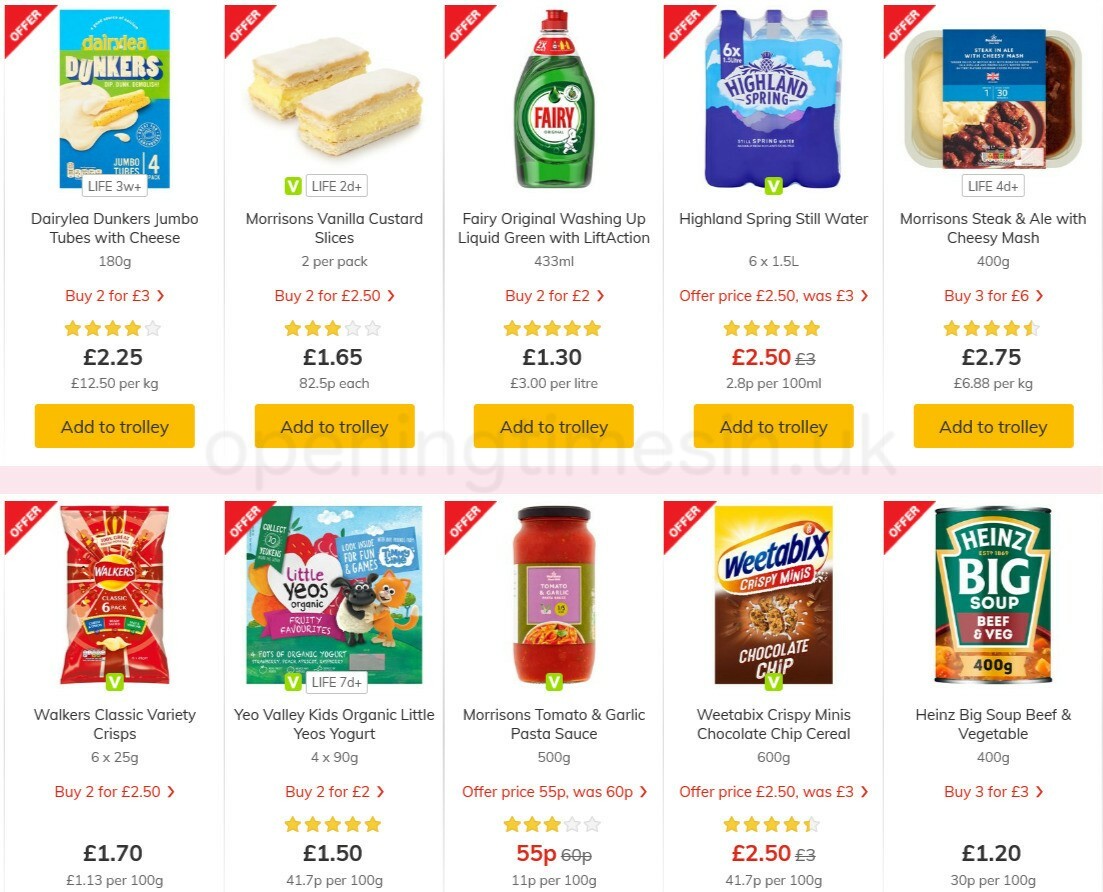This is a screenshot from what appears to be Amazon UK, displaying a selection of 10 different products. Each product is highlighted with a star rating system above the price, and a red triangle labeled "offer" in the top left corner of the product thumbnail.

In the top row:
1. **Dairylea Dunkers** - Jumbo tubes with cheese.
2. **Morrison's Vanilla Custard Slices**.
3. **Fairy Dish Washing Liquid**.
4. **Highland Spring Water**.
5. **Morrison's Steak and Ale with Cheesy Mash** - resembles a TV dinner.

In the second row:
6. **Walker's Classic Variety Crisps**.
7. **Yeo Valley Kids Organic Little Yeo's Yogurt**.
8. **Morrison's Tomato Garlic Pasta Sauce**.
9. **Weetabix Crispy Minis, Chocolate Chip Cereal**.
10. **Heinz Big Soup Beef and Vegetable**.

The prices for the products are listed as follows: £2.25, £1.65, £1.30, £2.50, £2.75, £1.70, £1.50, £0.55, £2.50, and £1.20 respectively. 

There are large, rectangular yellow buttons labeled "Add to Trolley" indicating their availability for online purchase.

Each product description includes details such as the weight (e.g., "6 x 25 grams") and specific offers like "2 for £2.50" or "3 for £3" for better clarity on discounts.